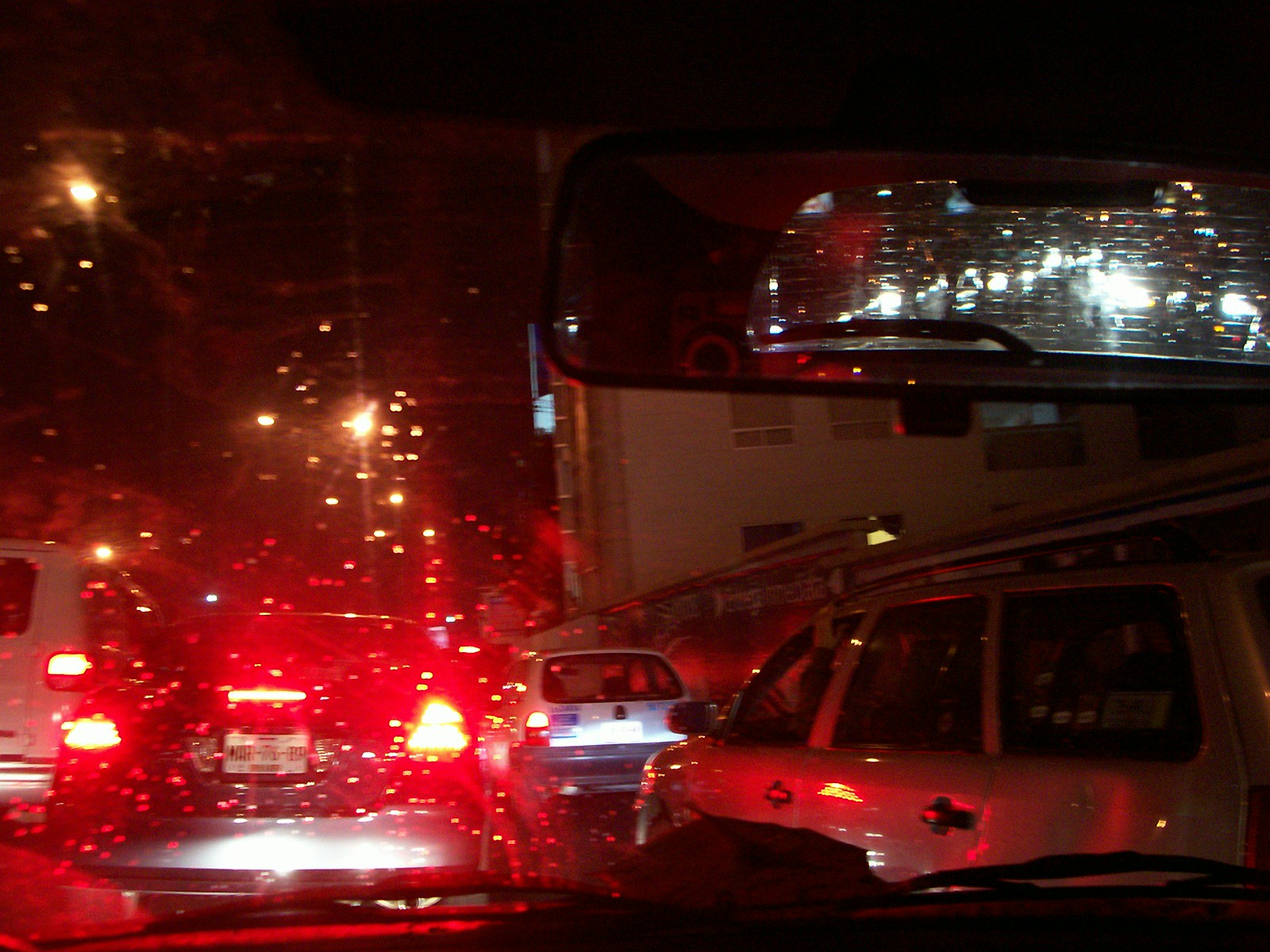A photograph captures a rainy city street from inside a car, the windshield dappled with raindrops and lit up by the red brake lights of the car ahead. To the right, a silver SUV with two doors and three windows stands parked, adjacent to a white car. On the right side of the frame, a multi-story white building looms. On the left, a white van with glowing red lights is visible, accompanied by a tree illuminated by a yellow streetlight. Another yellow streetlight stands prominently in the center of the scene. The rearview mirror reflects the bustling cityscape behind, featuring a myriad of white lights and towering buildings. The reflection also shows part of the photographer's camera and the outline of their head.